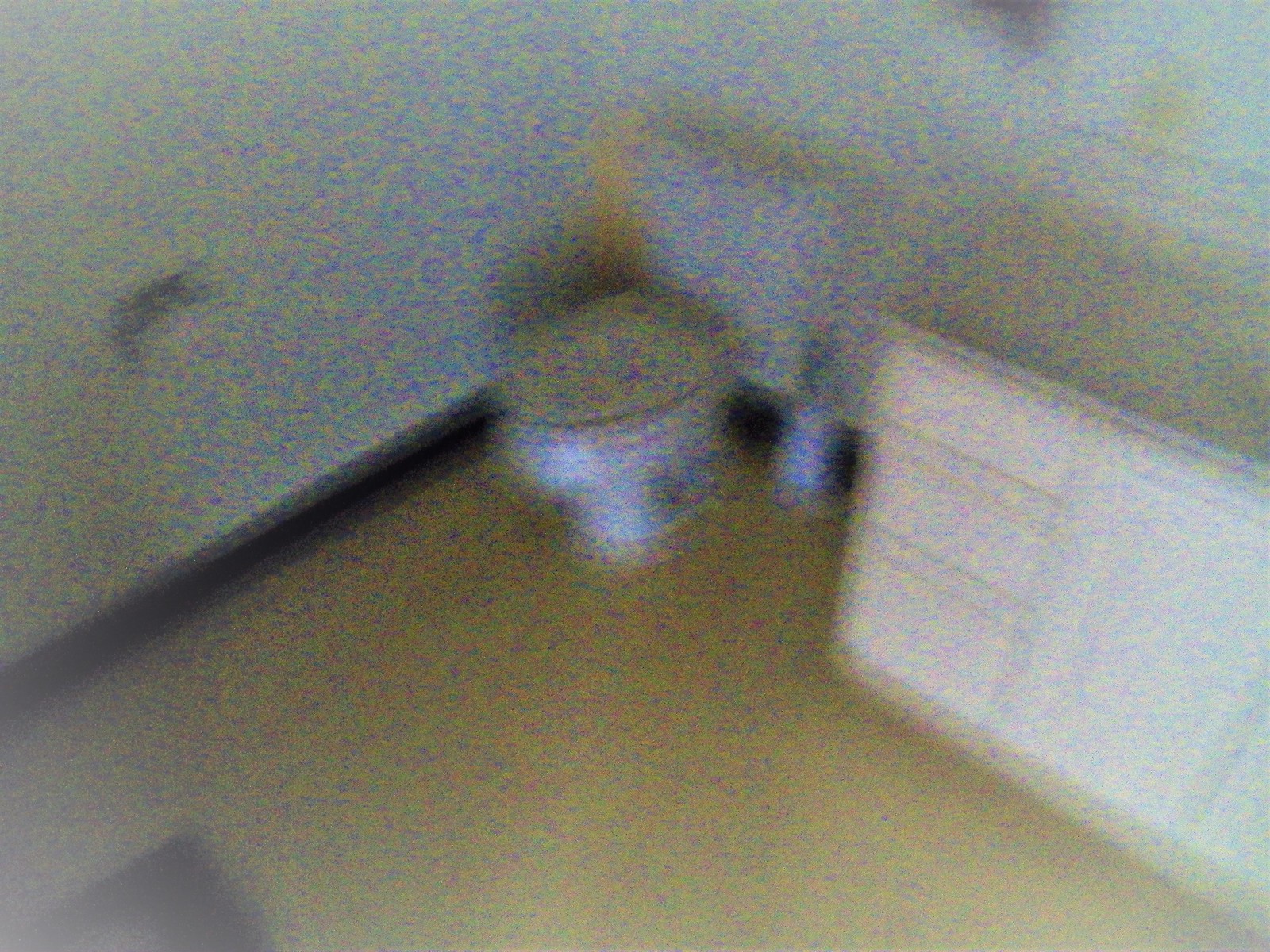The image depicts a blurry, low-resolution section of a bathroom with a very gloomy atmosphere. The focal point is a toilet with a white bowl and a yellow (or tan) closed top lid, situated on a yellow (or orange-tan) floor that has noticeable paint splatters in reds, blues, and greens. To the right of the toilet stands a brush holder, and further to the right, there's a white counter and multiple cabinets, including vertical drawers and an open door in the middle, all topped with a gray countertop. On the left side of the toilet, attached to the wall, is a toilet paper holder. The surrounding walls and the vanity feature a chaotic splash of colors including various shades of blue, purple, yellow, green, and splatter patterns that give the room a disorganized yet colorful appearance. Despite the blur and low resolution, the details convey an eclectic and vividly painted bathroom setting.